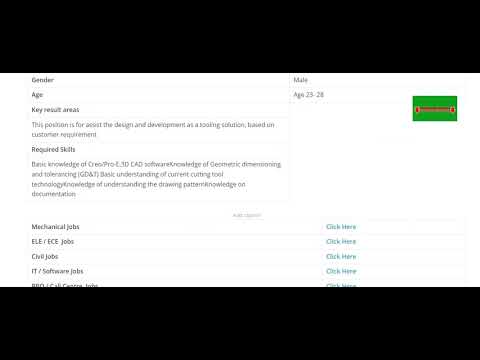This image shows a computer screen displaying a job description, although the text is slightly blurry and not entirely legible. The format includes black horizontal strips at the top and bottom, framing a white central area. The content is organized into columns. The left column lists attributes and requirements such as "Gender," "Age," "Key Result Areas," and "Required Skills," along with job categories like "Mechanical Jobs," "ECE Jobs," and "IT Software Jobs." Specific details to this position include "Gender: Male," and "Age: 23-28," indicating the desired candidate demographic. The job pertains to "Design and Development" based on customer requirements, with necessary skills including a basic knowledge of CAD software and an understanding of CAD technology. There is a notable green rectangle with a red line crossing through it in the upper right corner of the image. Multiple "Click Here" links are present at the bottom of the screen, one for each job category mentioned.